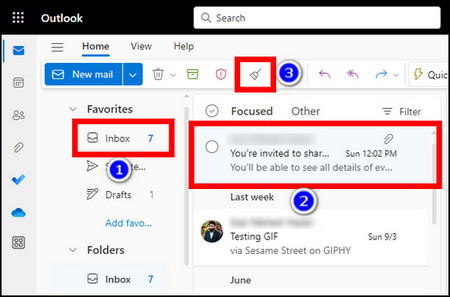The image depicts a small screenshot of an Outlook message search window. At the top, a black banner bar displays the name "Outlook" accompanied by a nine-dot icon, with a blank white search box adjacent to the title. Directly beneath this banner, the top menu bar offers three options: Home, View, and Help, with Home currently selected.

The menu bar below these options features various icons for navigating through Outlook. The first section, labeled New Mail, is highlighted in blue, and contains multiple icons. Prominently displayed is a blue circle with a white trim, enclosing the white number '3'. 

Below this section are two main columns: Favorites, and Focused and Other emails corresponding to the selected items in the first column. Under Favorites, the Inbox section, highlighted with a red outline, shows 'Inbox 7'. A smaller blue circle with the number '1' appears beneath the Inbox.

The second column under the Focused section, which is highlighted, shows a snippet of the first message, including a bold partial title with the day and time next to it. A paperclip icon indicates an attachment, circled in red, with a blue button numbered '2'. 

Above the main column, a navigation icon resembling a broom, likely for cleaning or sweeping, is circled in red with a blue button numbered '3'. Below the selected item, titles and snippets of other emails are visible, including a message titled "last week" and another titled "Testing at GIF" dated Sunday, September 3rd.